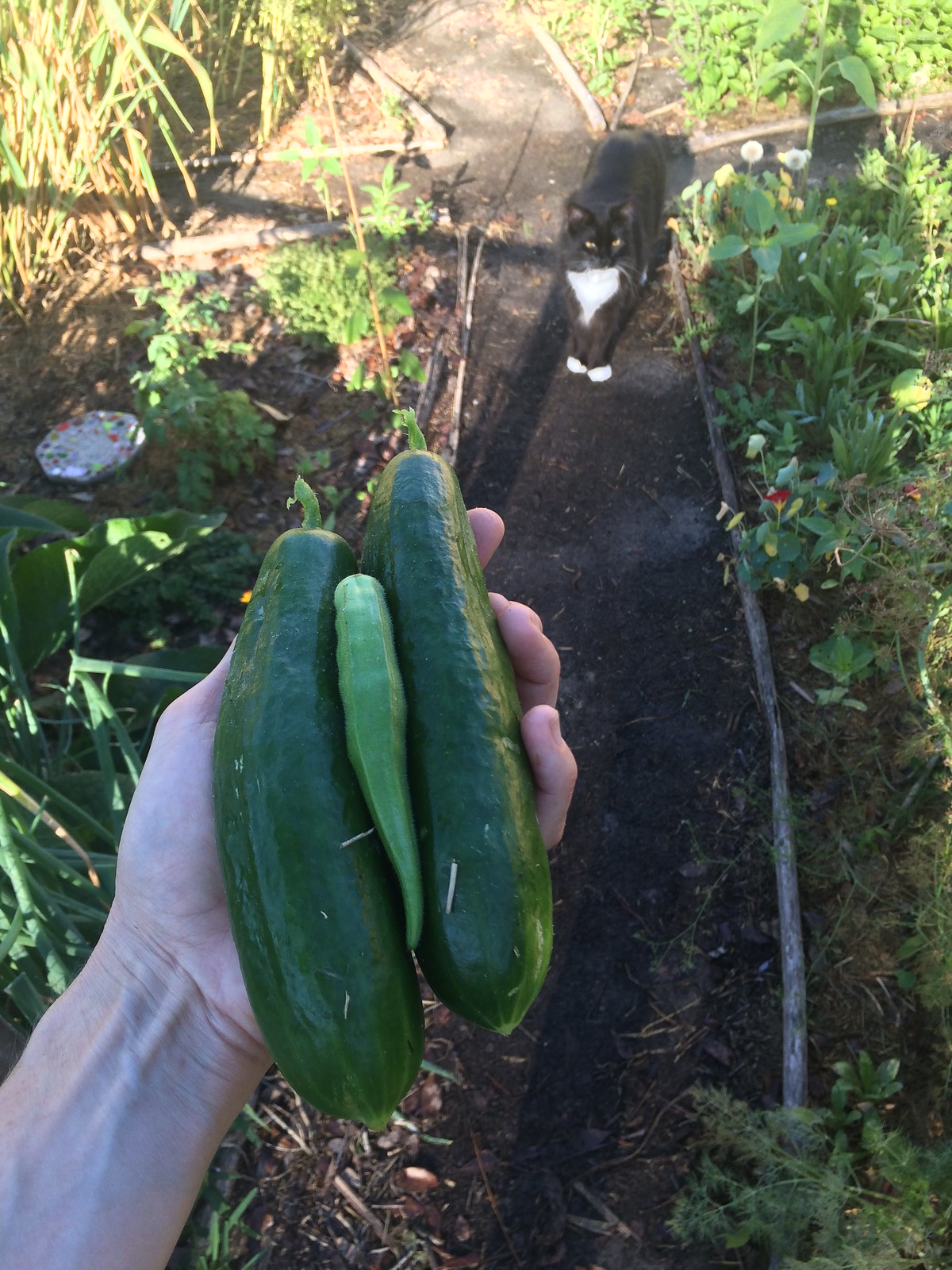In this detailed outdoor photograph, taken either in the early morning or late evening due to the long shadows cast, we see a lush garden setting filled with various green vegetation, including peppers, courgettes, and possibly lettuce. The garden paths, marked by dark soil and bordered with pieces of wood or bamboo, crisscross from north to south and east to west. At the center of the image, a serene black and white tuxedo cat with striking gold eyes, a large white triangle on its chest, and white paws gazes up towards the camera. Just above the cat, a Caucasian person’s left hand, with visible wrist tendons, extends into the frame, holding three cucumbers—two large dark green ones and a smaller light green one. The sun, positioned behind the photographer, bathes the top section of the photograph in light, accentuating the vibrant color of the garden. A whimsical white bowl with red, green, and blue dots is also visible on the ground amidst the leafy vines and plants, completing this picturesque garden scene.